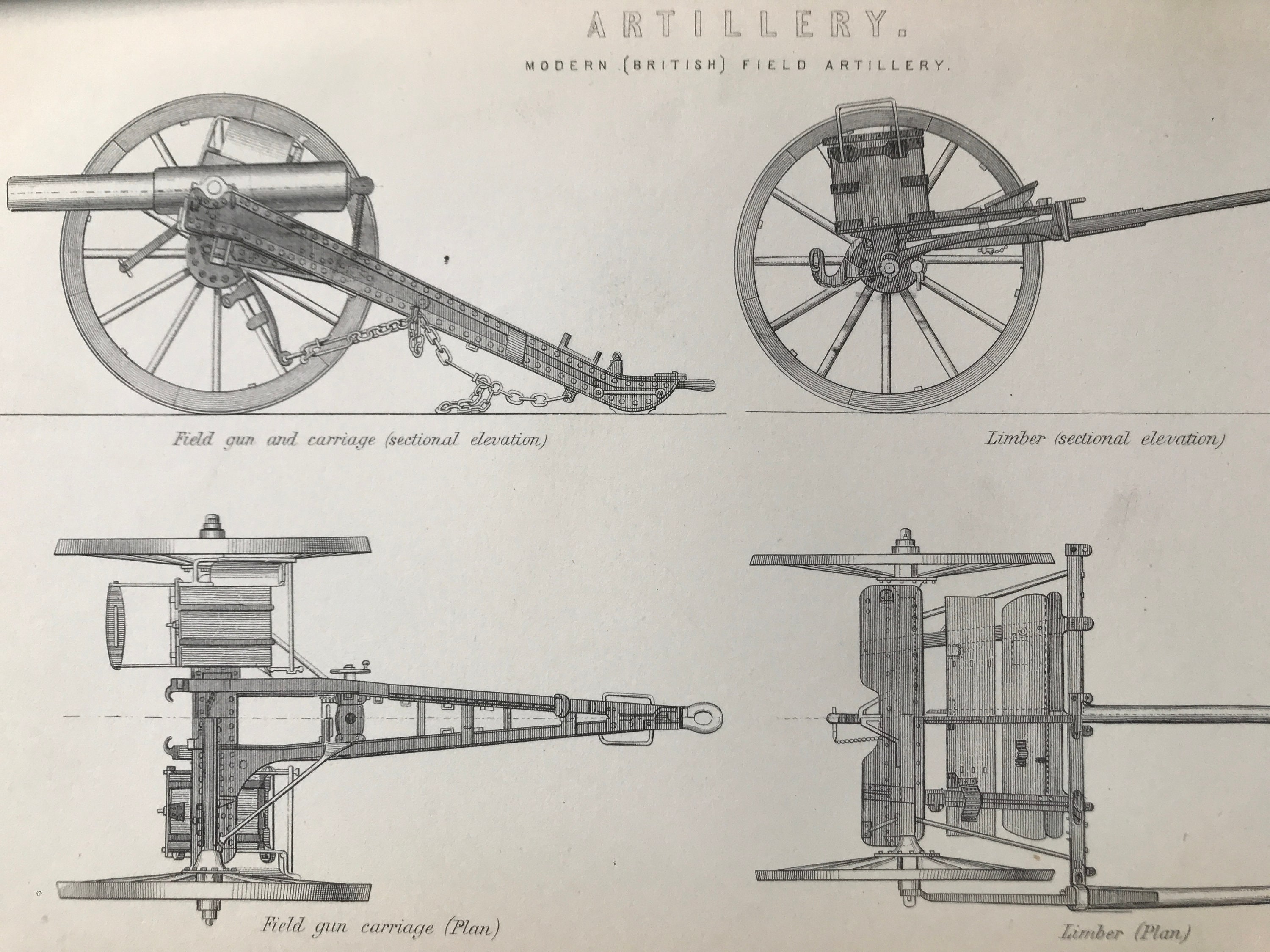This photograph captures an old, smudged, and faded diagram on paper, titled "Artillery Modern (British Field Artillery)" at the top. The diagram features four detailed drawings of artillery pieces. 

The top-left drawing, labeled "Field Gun and Carriage Sectional Elevation," depicts a large, cannon-like gun mounted on a giant wheel with a substantial support beam, showcasing a side view of the machinery. Beside it, on the top-right, is the "Limber (Sectional Elevation)" drawing, illustrating another large wheel with an attached box and an extending neck, positioned to show a sectional side view.

At the bottom left, the "Field Gun Carriage (Plan)" drawing provides a top-down view of the artillery, highlighting the two large wheels on either side, connected by a beam that resembles a crane extending from the middle. On the bottom right, the "Limber (Plan)" drawing, also presented in a top-down view, displays two wheels with connecting planks and an extension projecting off the page.

The diagram appears to showcase 19th-century British field artillery, emphasizing the intricate design and functionality of each part through detailed sectional and plan views.